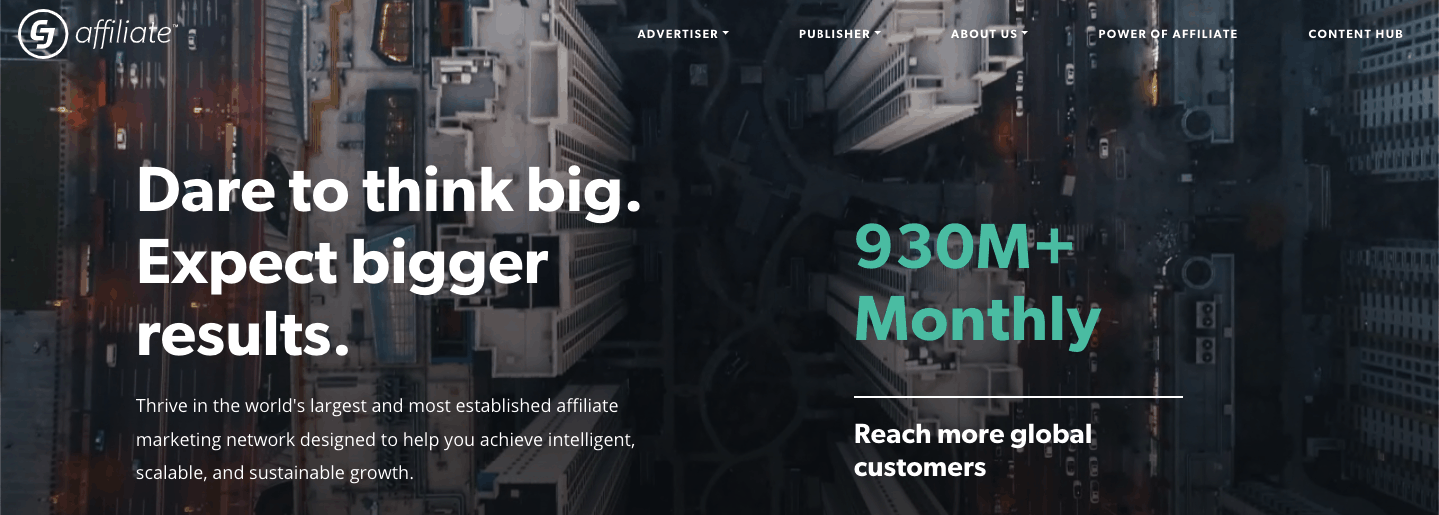This image is a detailed screenshot featuring a computer server room as the background. In the upper left corner, there is a white circle with the initials "CJ" inscribed within it. Adjacent to this circle, the word "affiliate" appears in lowercase, slightly italicized white letters. To the right of "affiliate," a menu displays the following options: "Advertiser," "Publisher," "About Us," "Power of Affiliate," and "Content Hub."

Positioned at the bottom left, a motivational slogan reads, "Dare to think big. Expect bigger results. Thrive in the world's largest and most established affiliate marketing network designed to help you achieve intelligent, scalable, and sustainable growth." To the right of this text, a prominent green message states, "930M+ monthly." Below this figure is a thin, horizontal white line, and further down, in white text, it reads, "Reach more global customers."

The screenshot is notably wider than it is tall and does not include any people, animals, birds, plants, flowers, trees, automobiles, or airplanes.